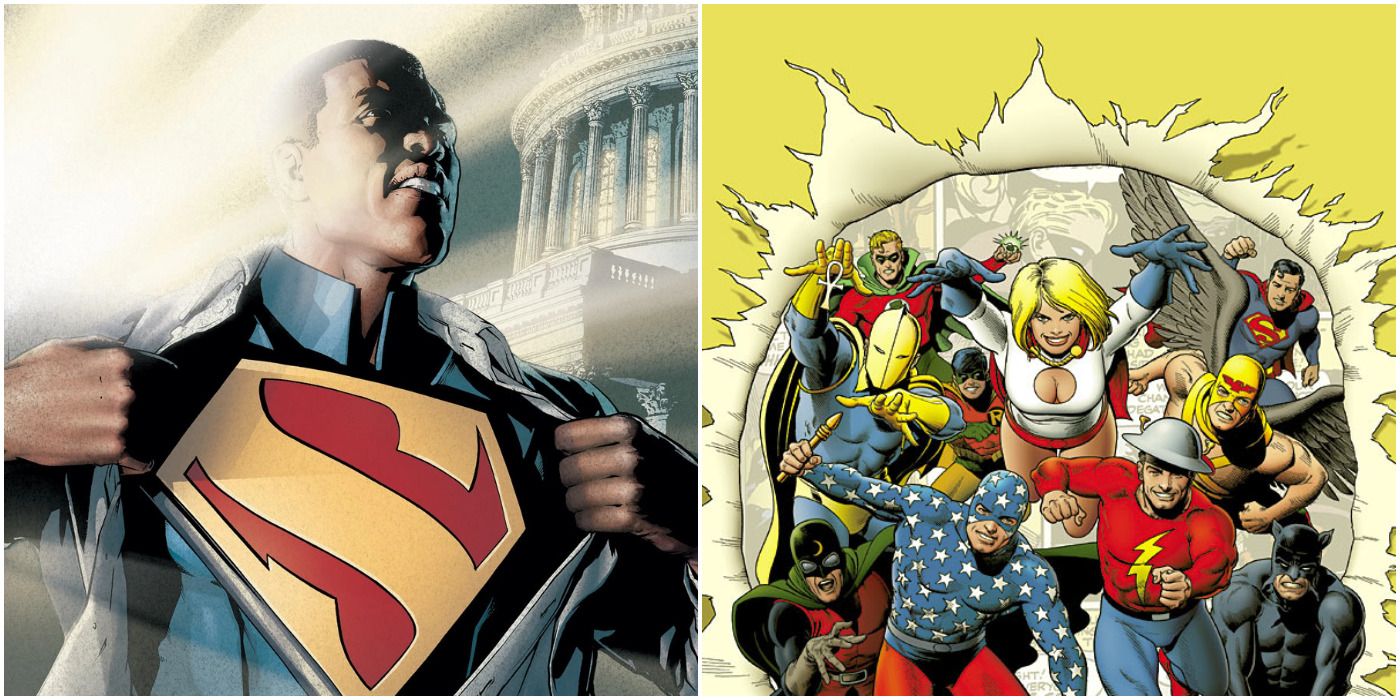The image features two side-by-side panels from DC Comics. The left panel depicts an alternate version of Superman, an African American who also serves as the President of the United States. Prominently featured, he is shown revealing his Superman logo—an iconic yellow 'S' on a red background—beneath his blue armor by unbuttoning his dress shirt. He stands resolute before the U.S. Capitol building, with beams of sunlight illuminating him from behind, symbolizing hope and power. This character dates back to an issue introduced around the year 2000.

The right panel bursts with vibrancy as iconic DC Comics superheroes seem to explode out of a torn yellow and beige paper backdrop. Leading this dynamic display is Power Girl, dressed in her distinctive white costume with a revealing chest cut-out, and complemented by a red skirt. Surrounding her are classic characters including the 1940s Flash in a red long-sleeved costume, blue pants, and a signature metal helmet; the original Green Lantern wearing a green cape over a red costume; and Dr. Fate, distinguished by his blue ensemble and gold helmet. Superman also makes an appearance in the background, while all the characters are depicted with jubilant expressions, highlighting their timeless and heroic spirits.